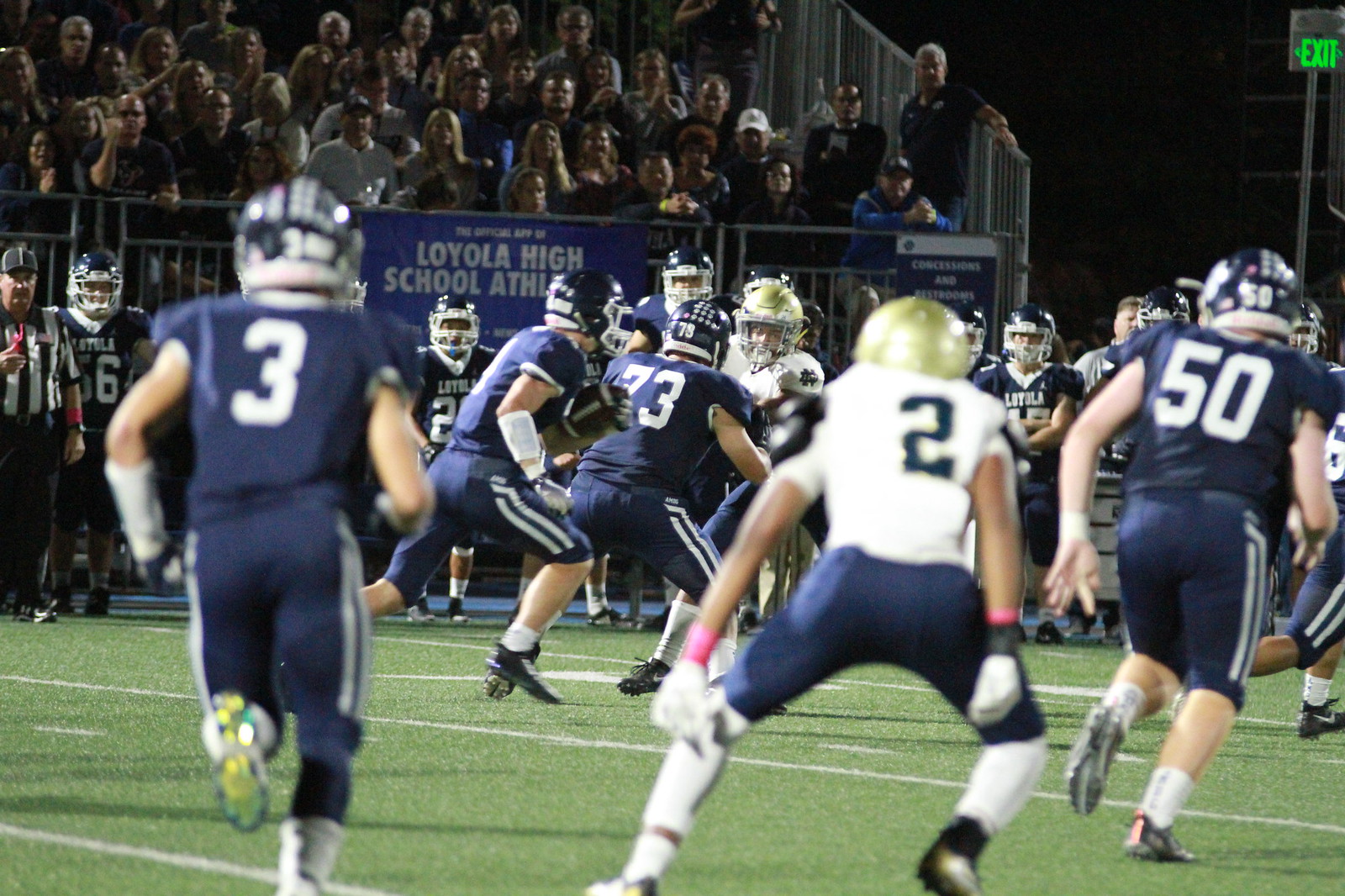The image captures a lively high school football game under the night sky, with powerful stadium lights illuminating the green turf field. The match features two teams: one team, currently in possession of the football, is clad in dark blue jerseys with white numbers and matching dark blue helmets, while their opponents wear white jerseys with dark blue numbers, gold helmets, and blue pants. Positioned on the left side of the image is a referee, easily identifiable in his black and white uniform, standing on the sidelines along with members of the dark blue team who are not on the field. 

Behind the action, the bleachers are packed with spectators, reflecting the excitement of a possible Friday night game. A prominent blue banner on the front railing of the bleachers displays "Loyola High School Athletics" in white text. The background is pitch black, highlighting both the illuminated field and the shadows cast by the players and the crowd. Additionally, a bright green exit sign is visible at the top right corner, adding to the details of the bustling scene.